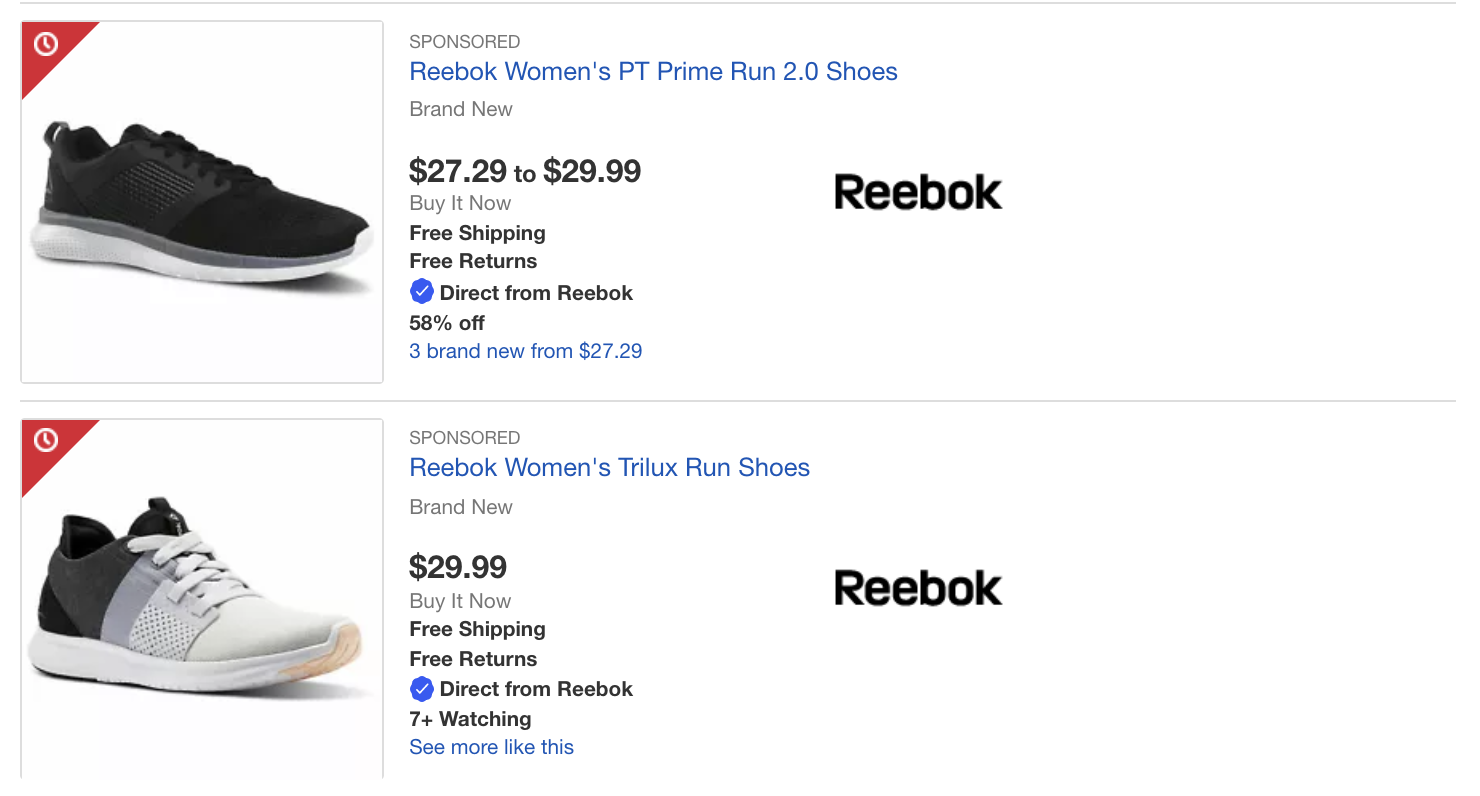This image is a screenshot of two sponsored advertisements for Reebok running shoes.

In the upper-left-hand corner of the first advertisement, there is a small red clock symbol. The featured shoe is primarily black, accented with a gray stripe above the sole, and a white sole. The text below the image reads: "Sponsored. Reebok Women’s PT Prime Run 2.0 Shoes. $27.29 to $29.99. Buy it now. Free shipping, free returns." A blue checkmark icon next to the text indicates that the item is "Direct from Reebok." A label at the bottom indicates the shoes are 58% off, with three brand new pairs available starting from $27.29. The Reebok brand logo is displayed on the right-hand side of the ad.

The second advertisement at the bottom also features a small red clock symbol in its upper-left-hand corner. The shoe in this ad shares a similar color scheme but with a different design. The area around the heel is black, transitioning into a medium gray stripe, followed by a light gray stripe with a mesh texture. The toe area is an almost white, very light gray, accented with a light peach or light orange color at the top. The sole is white, and the laces are white as well, unlike the black laces of the first shoe. The description reads: "Sponsored. Reebok Women's Trilex Run Shoes. Brand new. $29.99. Buy it now. Free shipping, free returns." It also includes a blue checkmark indicating "Direct from Reebok" and notes that there are 7+ people watching the item. The Reebok logo is displayed on the right-hand side of the ad.

Both advertisements prominently feature the Reebok brand and highlight the buying incentives such as discounts, free shipping, and free returns.